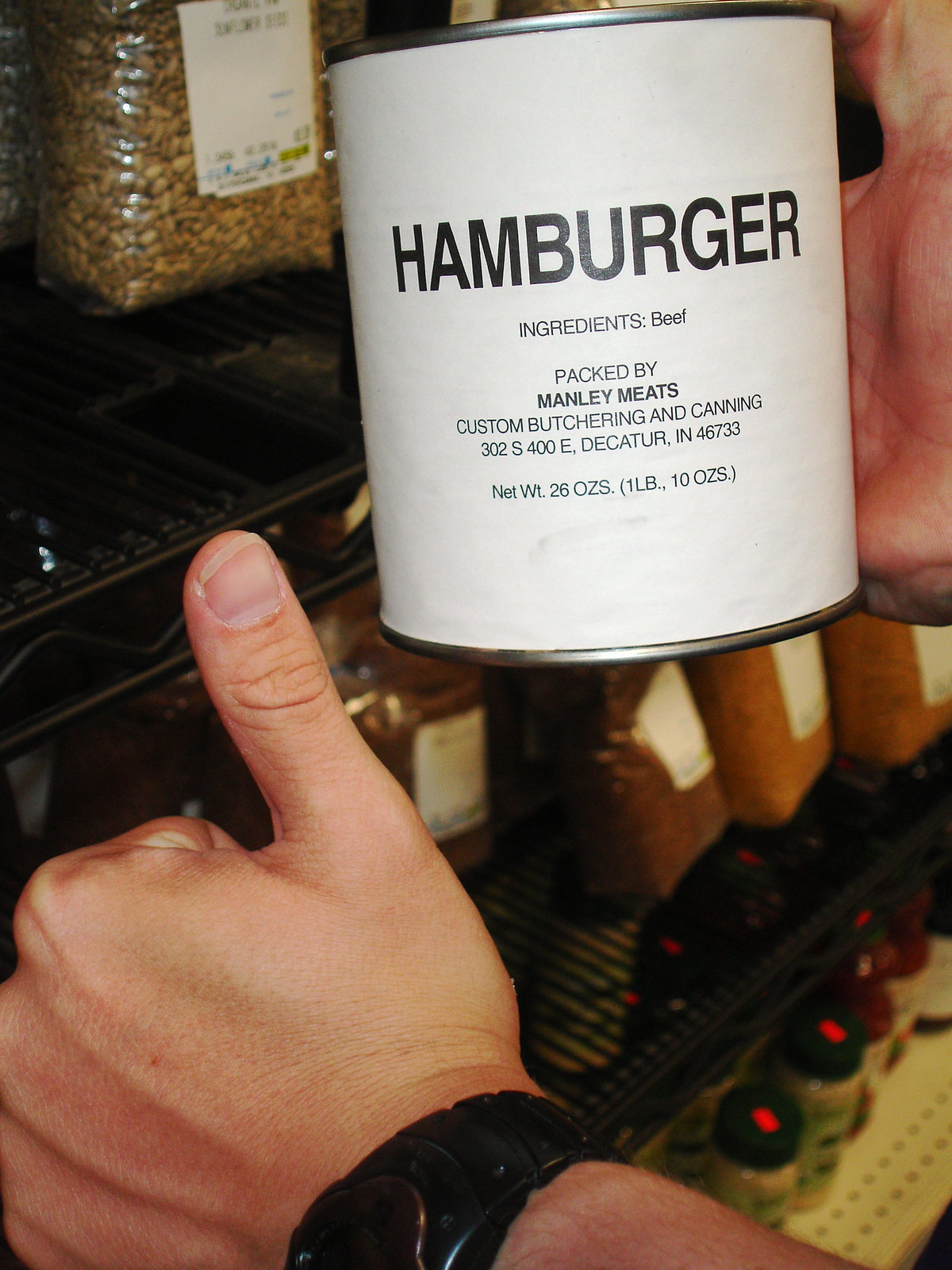In the image, a person is holding a can labeled "Hamburger," adorned with a white pepper leaf design. The can has an inscription that reads: "Ingredients: Beef, packed by Manly Meats, Custom Butchery and Canning, 302 S 400 E, Equator, Indiana, 46733," and notes its net weight as 26 oz, equivalent to 1 lb 10 oz. Nearby, on a black shelf, is a bag of nuts featuring a label and a visible price tag. Below this, another shelf displays various bagged items. At the bottom is a third shelf, lined with crispy goods and items featuring black lids with orange stickers. Additionally, there are jars of unidentified contents.